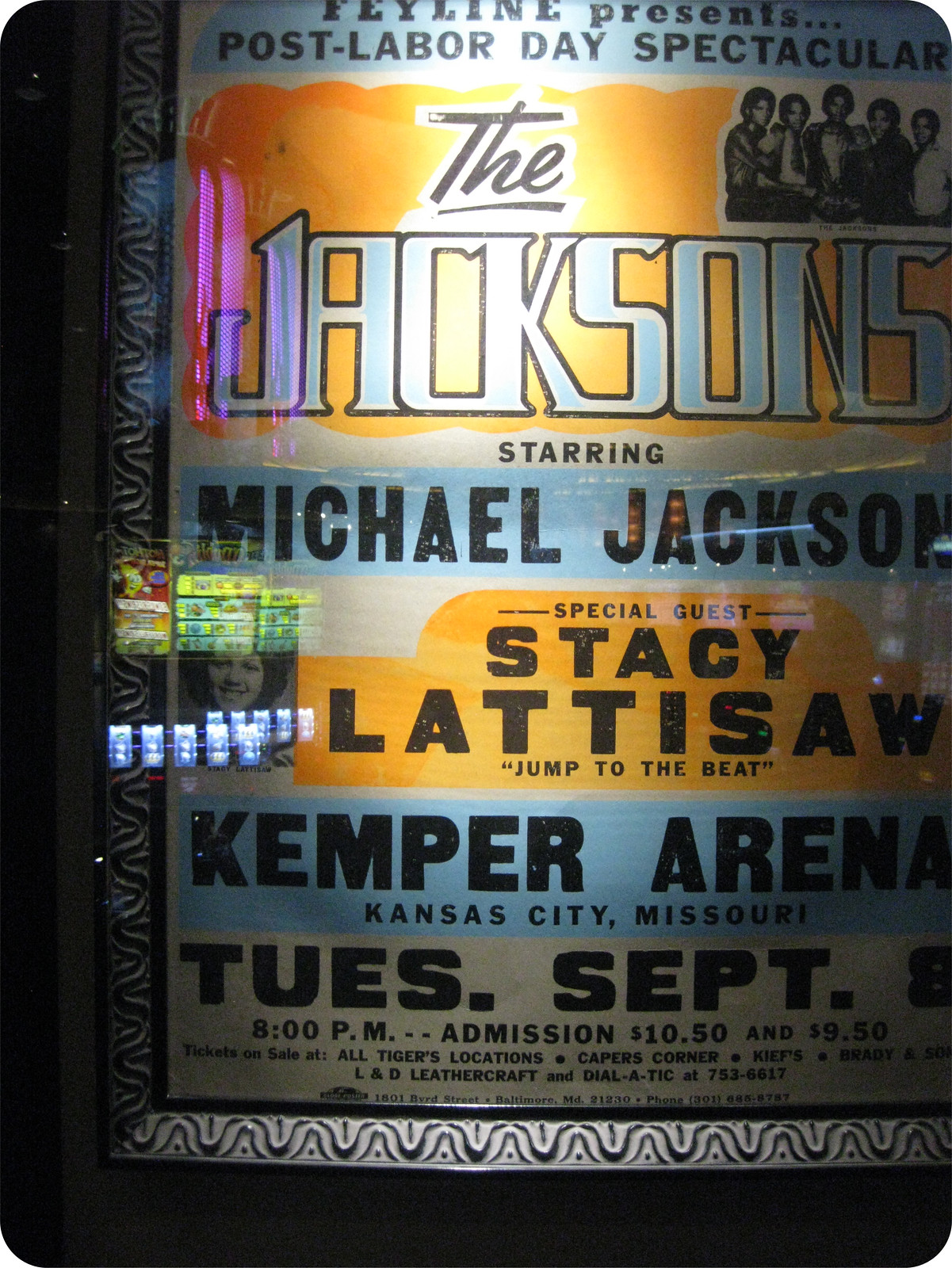In this image, we see a poster advertising a concert for The Jacksons, featuring Michael Jackson. The event, billed as the "Post-Labor-Day Spectacular," is presented by Fae Line and will take place at the Kemper Arena in Kansas City, Missouri, on Tuesday, September 8th, at 8 p.m., with admission prices of $10.50 and $9.50. Special guest Stacy Lattisaw is also highlighted on the poster. 

The poster prominently features the band's name "The Jacksons" in large blue letters on a yellow background, and includes a smaller black-and-white picture of the Jackson family. The text on the poster is mostly in black, set against alternating backgrounds of yellow and blue. Details about ticket sales are provided, including locations such as All Tigers Locations, Capers Corners, Keefs, Brady and Sons, L&D Leathercraft, and a contact number for Dial-A-Tick. 

Encased behind glass and slightly off-centered to the right, the poster takes up nearly the entire width of the photo. The setting appears to be a dark room, potentially an exhibit space, giving it a nighttime ambiance. The vivid colors of black, silver, gray, blue, yellow, purple, green, and orange further enhance the vibrant and nostalgic feel of the poster.